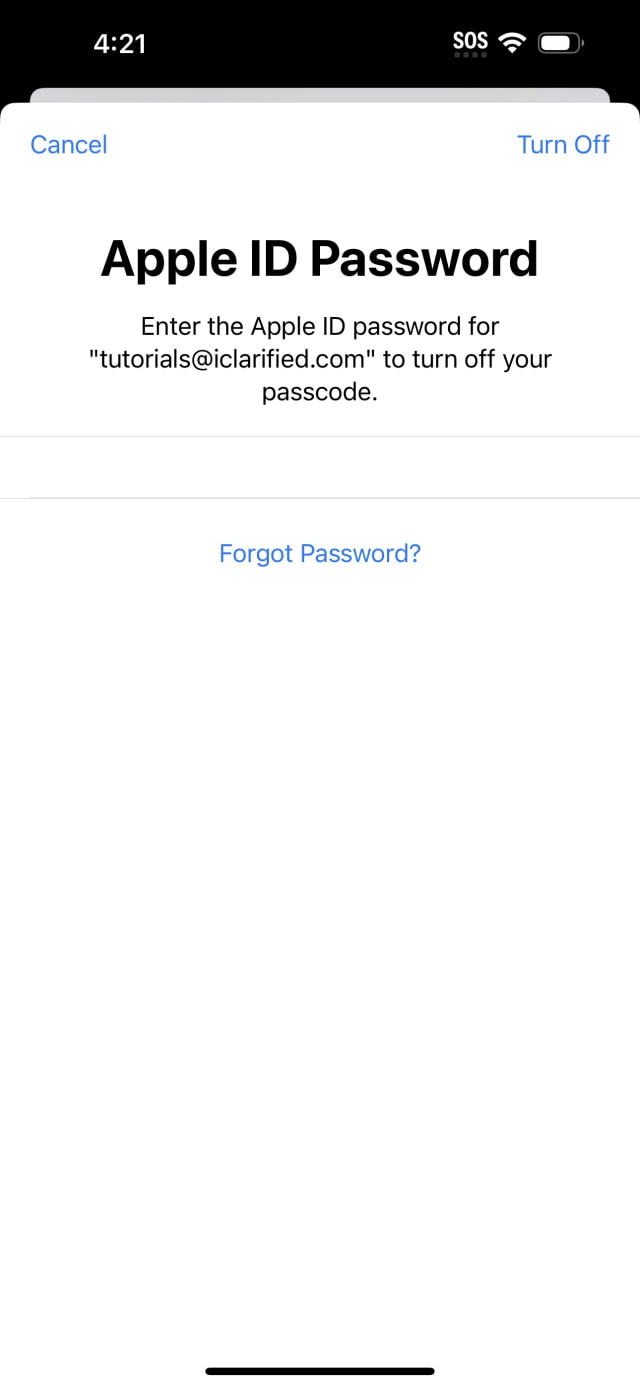A cell phone screenshot displays the "Sign In to Your Apple ID" interface. At the top of the image, a black bar spans from left to right. On the upper left-hand side of this bar, the time is displayed in white font as "4:21." On the upper right-hand side, the status indicators show "SOS," a fully connected Wi-Fi icon, and a battery icon.

Below this, a white block section contains navigation options. In the top left corner of this block is a "Cancel" button, while the top right corner features a "Turn Off" button. Beneath this line, there is a space followed by a bold, large-font heading that reads "Apple ID Password."

Further down, there is a smaller-font instruction: "Enter the Apple ID password for tutorials@iClarify.com to turn off your passcode." At the bottom, a hyperlink labeled "Forgot Apple ID or password?" is available for users needing assistance with their login credentials.